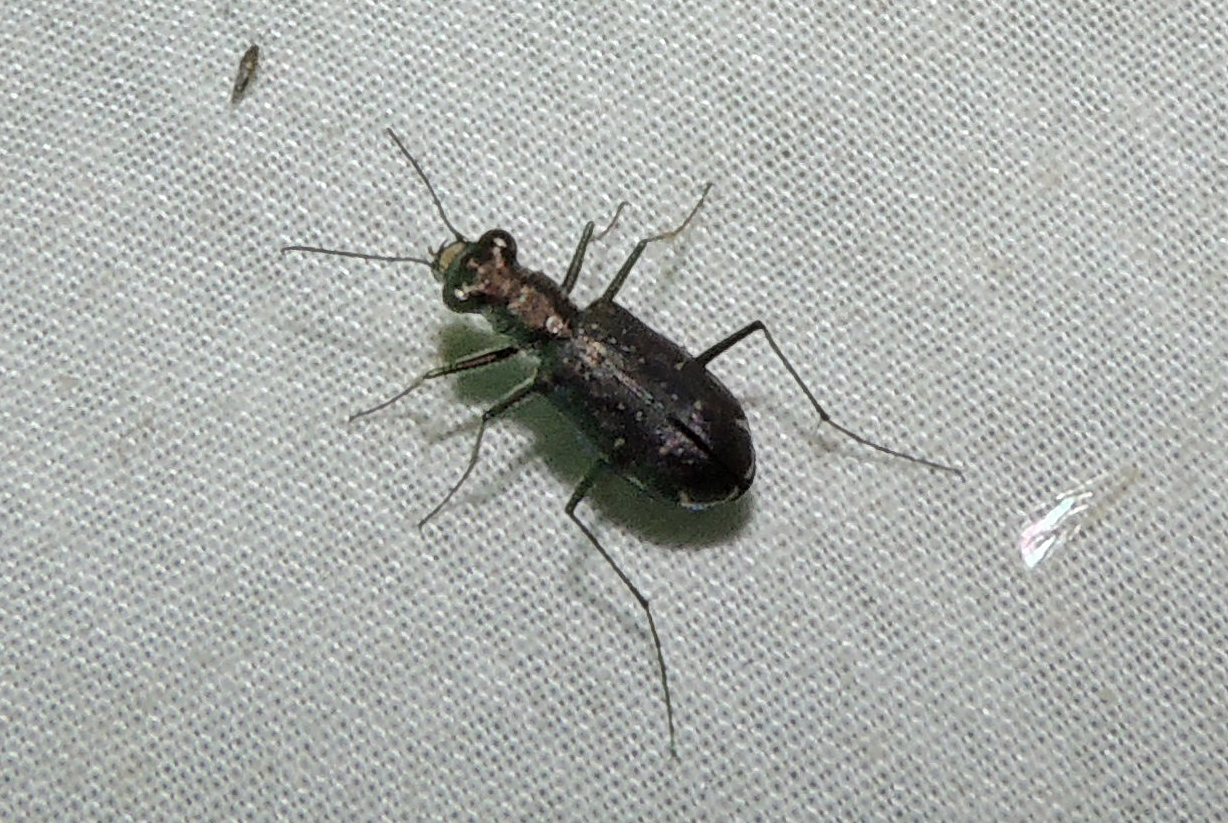The image captures an extreme close-up of a large bug perched on a white, finely stitched piece of fabric, possibly a sheet or pillowcase. The bug, which exhibits a glossy black color with some white speckling, has a pill-shaped body and a narrow, oval-shaped abdomen. Its head features bulging, circular eyes on either side, and two very long, thin antennae. The bug's six legs are spindly, with the front pair shorter and the back pair notably longer. Its wings are beetle-like and black, giving it a resemblance to a beetle, though it could be mistakenly identified as a different type of insect due to its unique features. The scene includes what appears to be a piece of clear plastic or a wing close to the bug's right leg, and a tiny bug is visible in the upper left corner of the image.